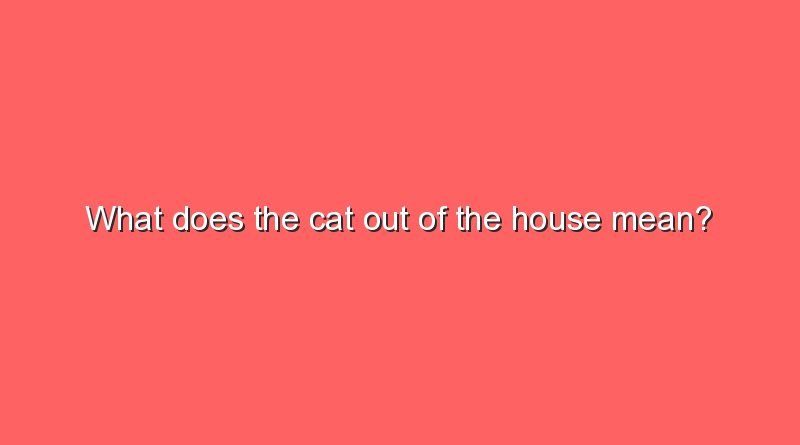The image displays a large, horizontally-oriented rectangle in a salmon pinkish-red color. Centrally positioned within the rectangle is a line of text that reads, "What does the cat out of the house mean?" The first letter of the text is capitalized, while the rest are in lowercase. The text is white with a black outline and a subtle black shadow behind each letter, giving it a slightly three-dimensional effect. The background is smooth with pointed edges, and no other elements or lines distract from the central question, making the overall presentation simple and clean.